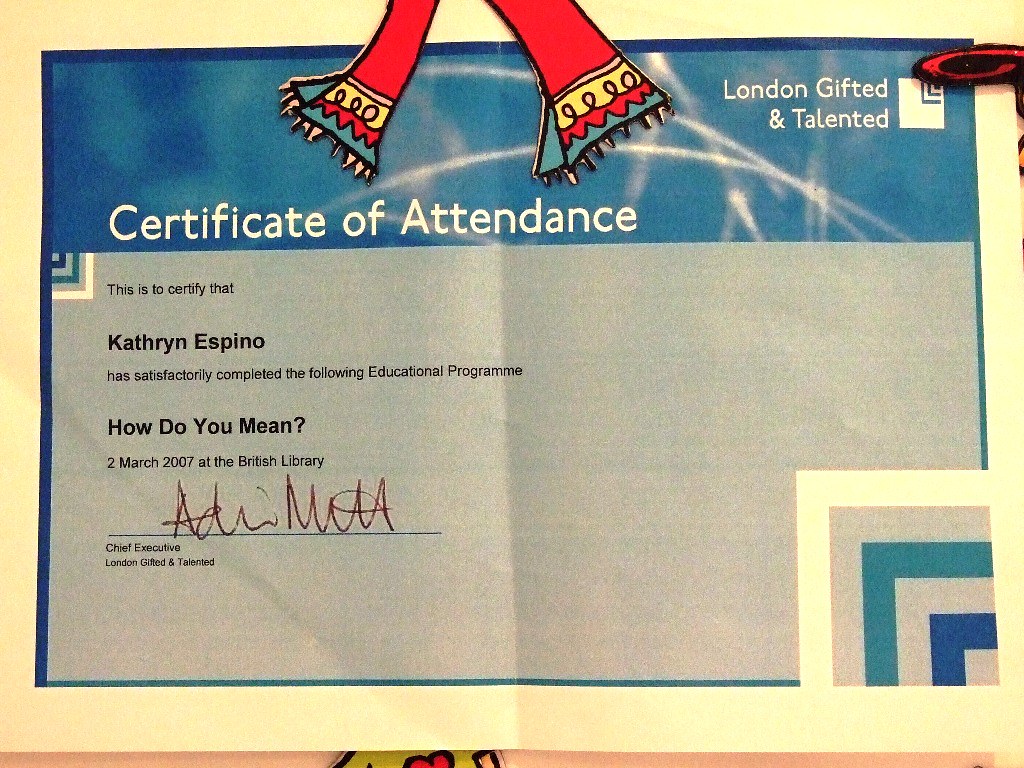The image depicts a Certificate of Attendance, prominently titled in white letters on a blue banner at the top. On the top right, "London Gifted and Talented" is inscribed. The certificate acknowledges that Catherine Espino has satisfactorily completed an educational program at the British Library, dated 2nd March 2007. A signature in red pen from the Chief Executive of London Gifted and Talented is also present. A notable feature is a red, yellow, and green scarf draped over the certificate, partially out of the frame. The bottom right corner of the certificate includes a pattern with white, gray, and blue elements, resembling a square with different colored stripes. The certificate has a yellow border and appears to be resting on a surface with additional out-of-focus papers or items around it.